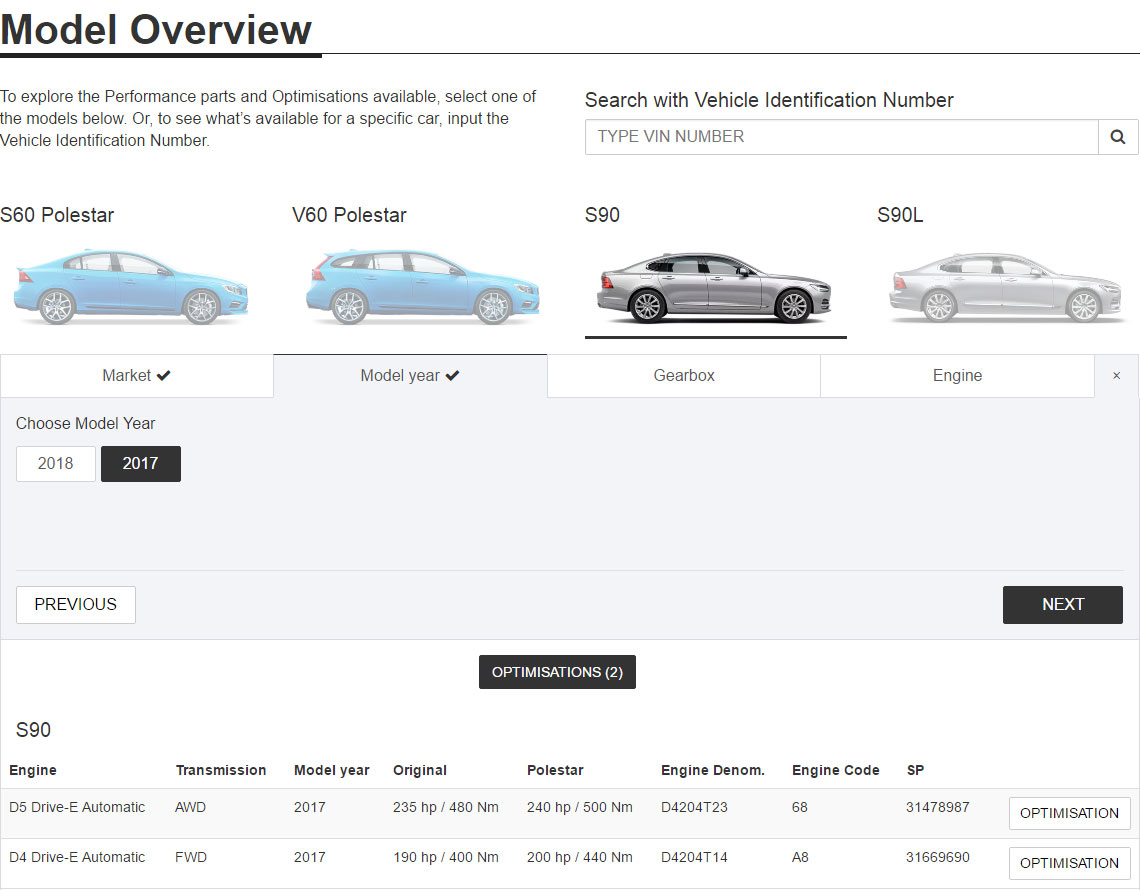The image's top left corner features the text "Model Overview" in black letters, highlighted by a bold underline. Just beneath this heading, the following instructions are provided: "To explore the performance parts and optimizations available, select one of the models below, or to see what's available for a specific car, input the Vehicle Identification Number."

To the right of these instructions is a search bar, labelled "Search with Vehicle Identification Number." Inside the search bar, it prompts users to "type VIN number," and a magnifying glass icon is present to initiate the search.

Below the search instructions, several vehicle models are displayed. The first vehicle is a blue S60 Polestar, followed by another blue vehicle, a V60 Polestar. The next vehicle displayed is a gray/silver S90, and subsequently, another silver vehicle, an S90L. Among these, the silver S90 appears to be the currently selected model.

Each vehicle has a set of details listed below it: "Market," "Model Year," "Gearbox," and "Engine." There is also an option to choose the model year, with 2018 and 2017 available, and 2017 currently selected.